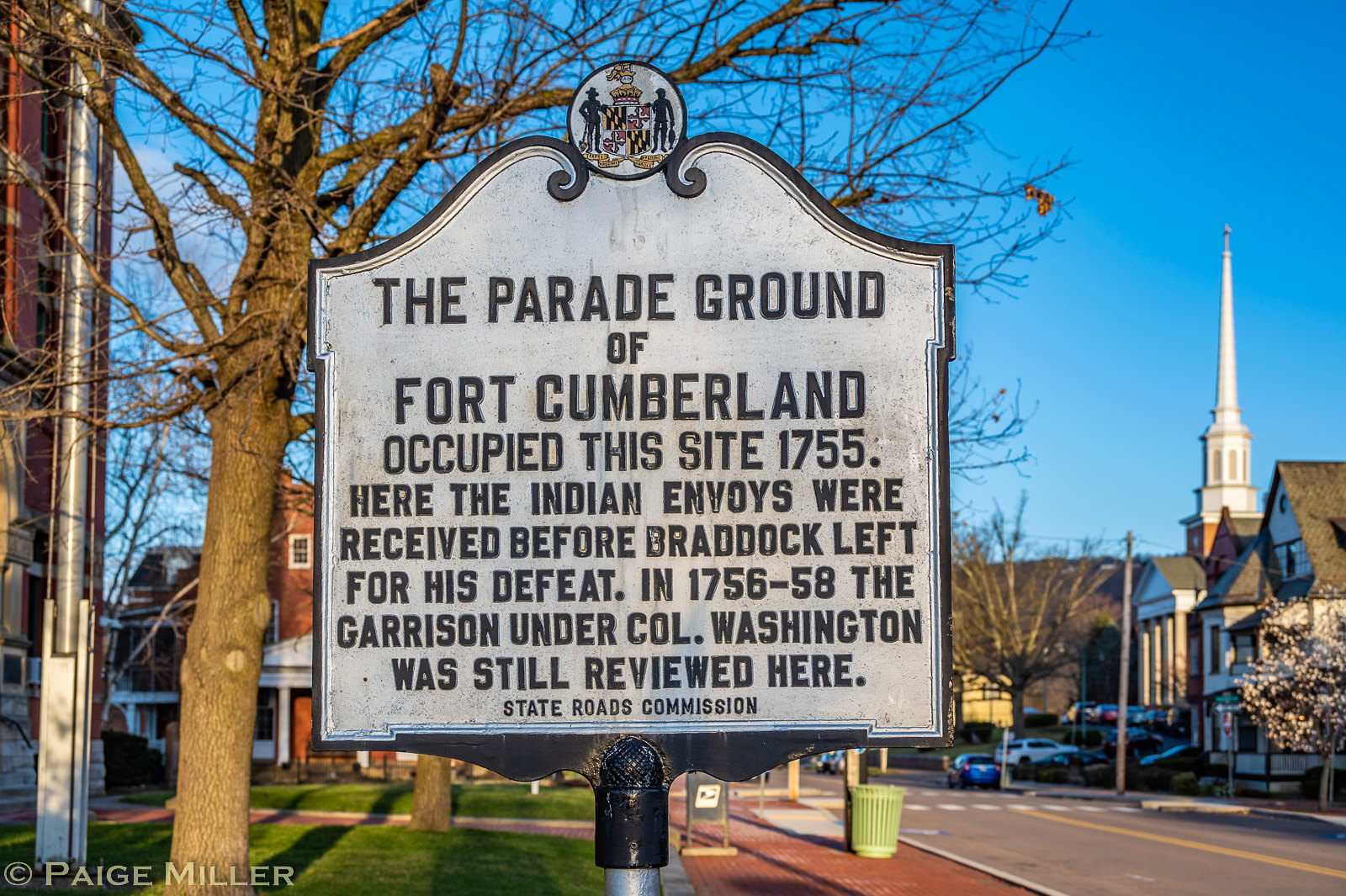The image is a daylight color photograph of a historic sign located in a small town. The sign, which is somewhat weathered and off-white, is edged in black and features a circle at the top with the Maryland state logo—a shield displaying black, yellow, white, and red elements—flanked by the silhouettes of two men. One of these figures appears to be wearing a cowboy hat. Black text on the sign reads:

"The parade ground of Fort Cumberland occupied this site in 1755. Here the Indian envoys were received before Braddock left for his defeat in 1756-58. The garrison under Colonel Washington was still reviewed here."

Below this, in smaller black text, it reads: "State Roads Commission." The sign is supported by a black pole with a silver brace, and the bottom left corner bears a transparent copyright mark for Page Miller.

In the background to the right, a tall white building with columns and a prominent steeple stands out, along with several parked cars, including a noticeable white car. To the left, a large tree with knobby branches and no leaves is visible, as well as partly obscured brick buildings. A clear blue sky completes the scene, with a street featuring double yellow lines and a crosswalk in the lower center of the image. Utility poles and a green trash can can also be seen in the background.